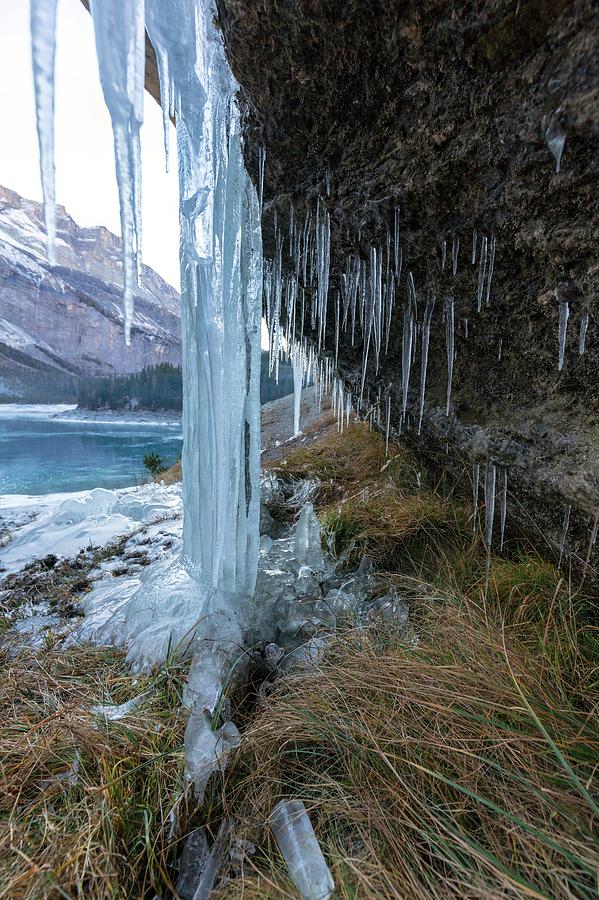The image showcases a winter nature landscape featuring a prominent rock overhang or cliff face on the right side. Hanging from this overhang are numerous sharp, long icicles, including a particularly large one that extends from the top of the rock all the way down to the ground, where ice has pooled. Some of the icicles have broken off and are scattered around. The ground beneath the rock face is covered in tall, brownish-green grass, indicating it is not heavily snow-covered. In the left background, a lake is visible, adding to the serene winter scene. Surrounding the lake, patches of snow dot the ground, and behind it, a picturesque mountain with snowy sections stands tall. The entire scene is framed by trees and a natural winter atmosphere.